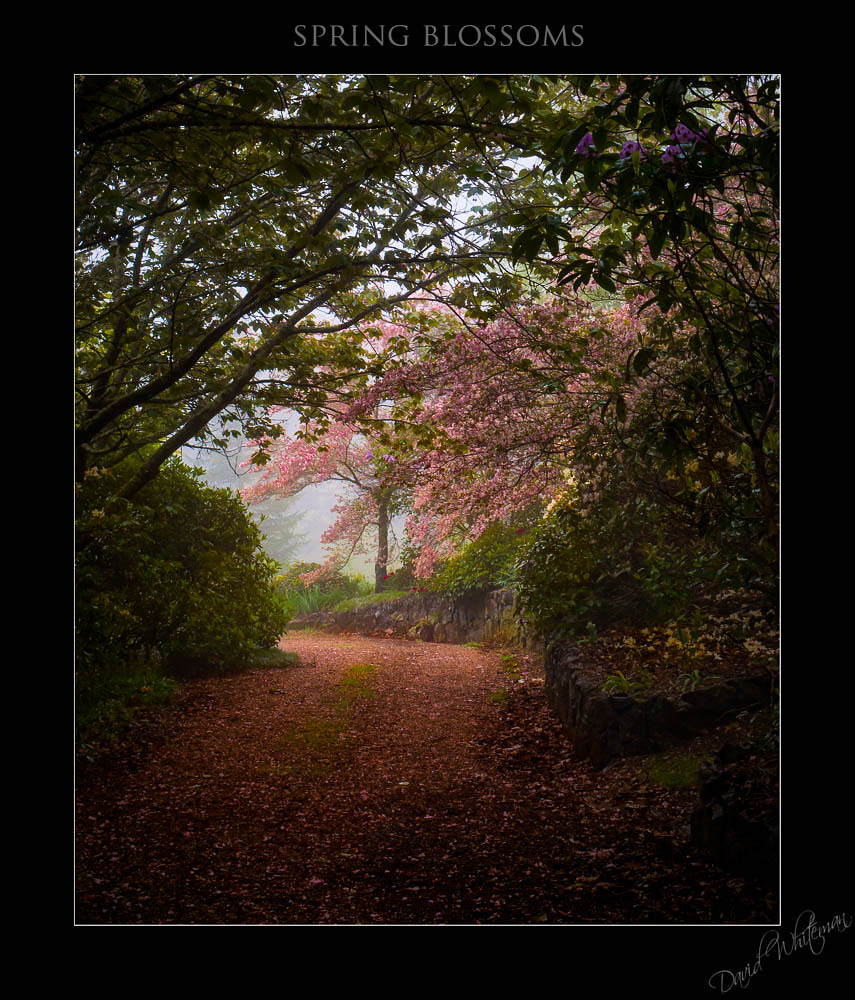The image features a beautifully detailed nature scene bordered by a thick, all-black frame with a thin white line along the edges. Across the top of the frame, the words "Spring Blossoms" are written in white. The centerpiece of the photograph is a serene, worn path flanked on either side by green trees. The ground of this trail is littered with fallen leaves, varying from shades of brown to delicate hints of pink. The path leads towards a bright light source in the distant background, where the sunlight pierces through the verdant canopy. Pink blossoms adorn the trees in the background, adding vibrant splashes of color against the predominantly green foliage and shadowy undertones. To the right of the path, there's a small rocky area, contributing to the scene's natural texture. At the bottom right corner, a cursive signature reads David P. Whiteman, although the last name is somewhat indistinct. This enchanting photograph, embodying the essence of spring, showcases a harmonious blend of shadow and light, with a culminating focus on the nature trail lined with blossoming trees.